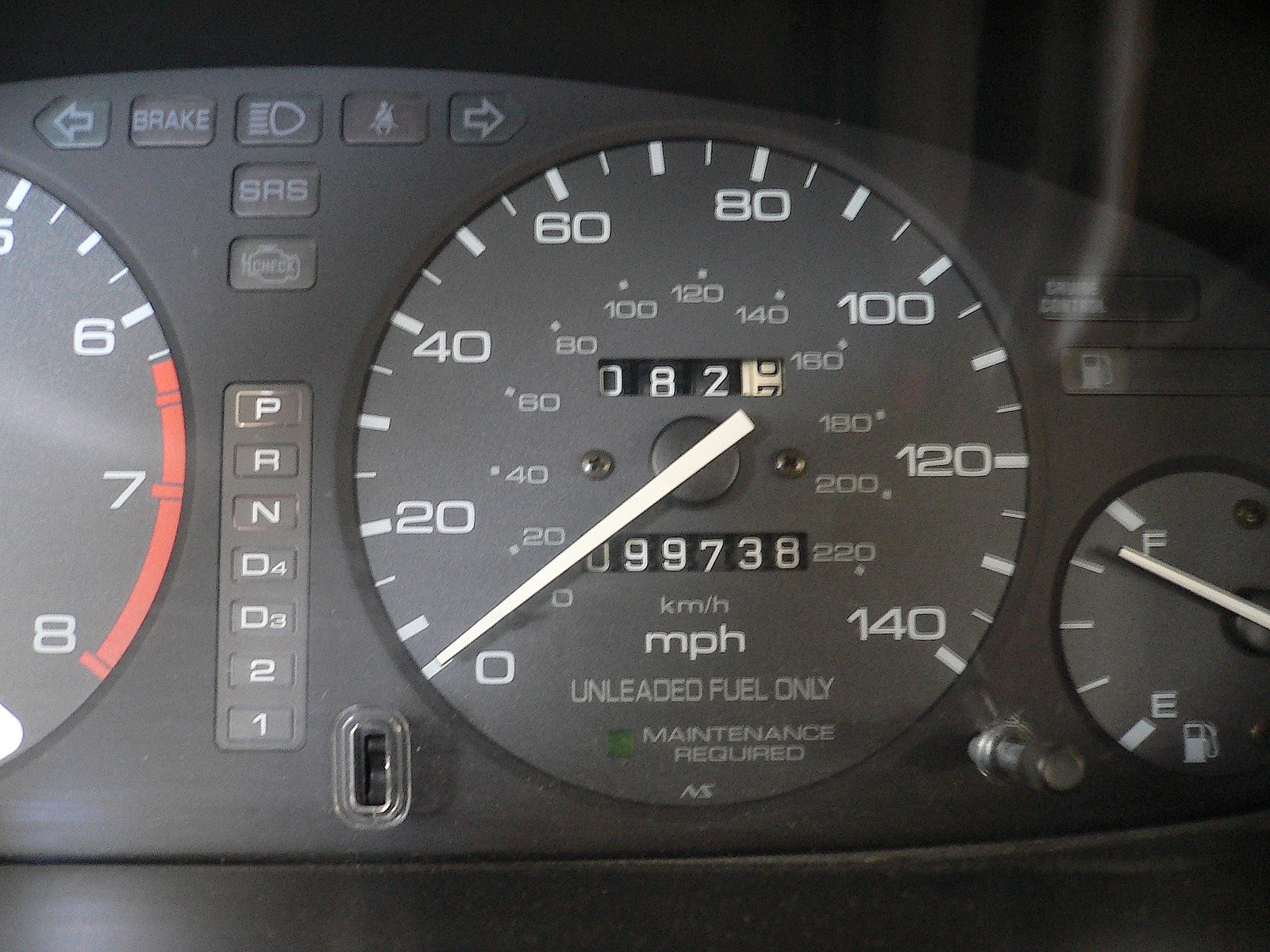A close-up photograph of a car's dashboard, prominently featuring the speedometer, which shows the vehicle has 99,738 miles on it. The speedometer dial, calibrated from 0 to 140 miles per hour, is clearly visible and includes a note stating "Unleaded Fuel Only." Surrounding the speedometer are various other indicators and buttons, beginning with a partially visible dial on the left. Adjacent to this is a cluster of indicator lights for the left and right turn signals, brake, check engine, seatbelt, and headlights. Below these, a gear mode display shows options for Park, Reverse, Neutral, and Drive. Additionally, there is a maintenance indicator light near the speedometer. On the far right, the fuel gauge displays the tank as approximately 80% full. The composition of the image captures a comprehensive view of the car's essential dashboard instruments and indicators.